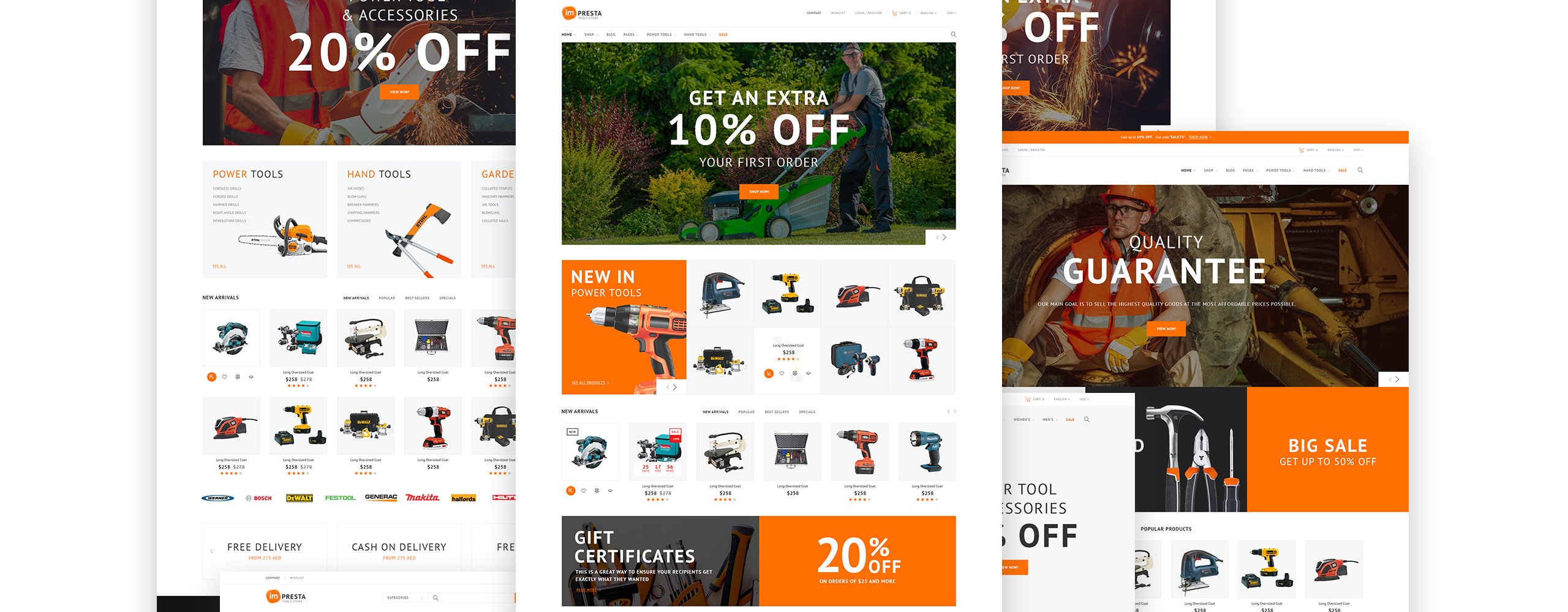This image features a collage of four overlapping screenshots, each showcasing various outdoor tools and carpentry equipment, reminiscent of a magazine layout. The top of the image displays a large picture of a worker wearing an orange hard hat, a reflective orange vest, gloves, and sleeveless attire, sitting in front of a massive tractor tire. Below this main image, several smaller images and product promotions are neatly arranged, advertising discounts of up to 20% off on various tools such as drills, hammers, and pliers. The upper section of the webpage visible in the screenshot prominently displays a "Quality Guarantee" banner, adding assurance to the advertised deals. Some text is partially obscured due to the overlapping nature of the screenshots, but the focus on quality outdoor tools and carpentry items is unmistakable.